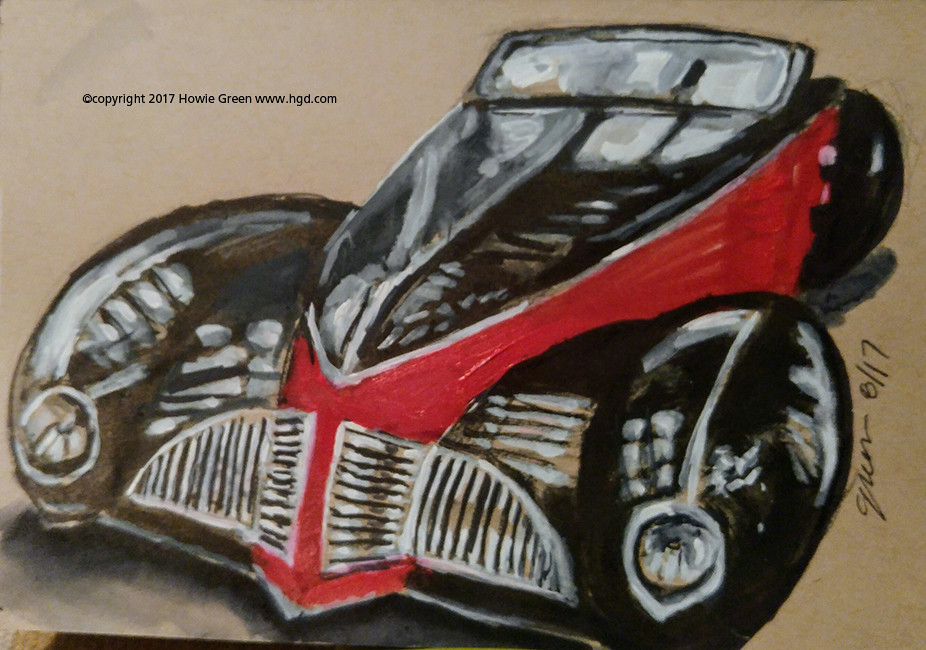This detailed illustration, which appears to be an acrylic painting or possibly pastel on toned paper, features a highly rendered, futuristic-looking sports car. The dynamic vehicle boasts a bright red and black chassis, wrapping around a sleek yet compact body. The car contrasts its wide front, resembling a hoverboard, with its increasingly narrow back, evoking a sailboat's taper. The front end includes a chrome-like grille, two headlights, and a low-profile windshield, and the design integrates black wheel wells around a single black back tire, suggesting a three-wheeled design with two front tires. The artist has expertly applied highlights to enhance the metallic look of the car, with shadows beneath creating depth. Signed "Galan 817" in the bottom right corner, the artwork is copyright 2017 Howie Green, with www.hgd.com listed in the upper left.